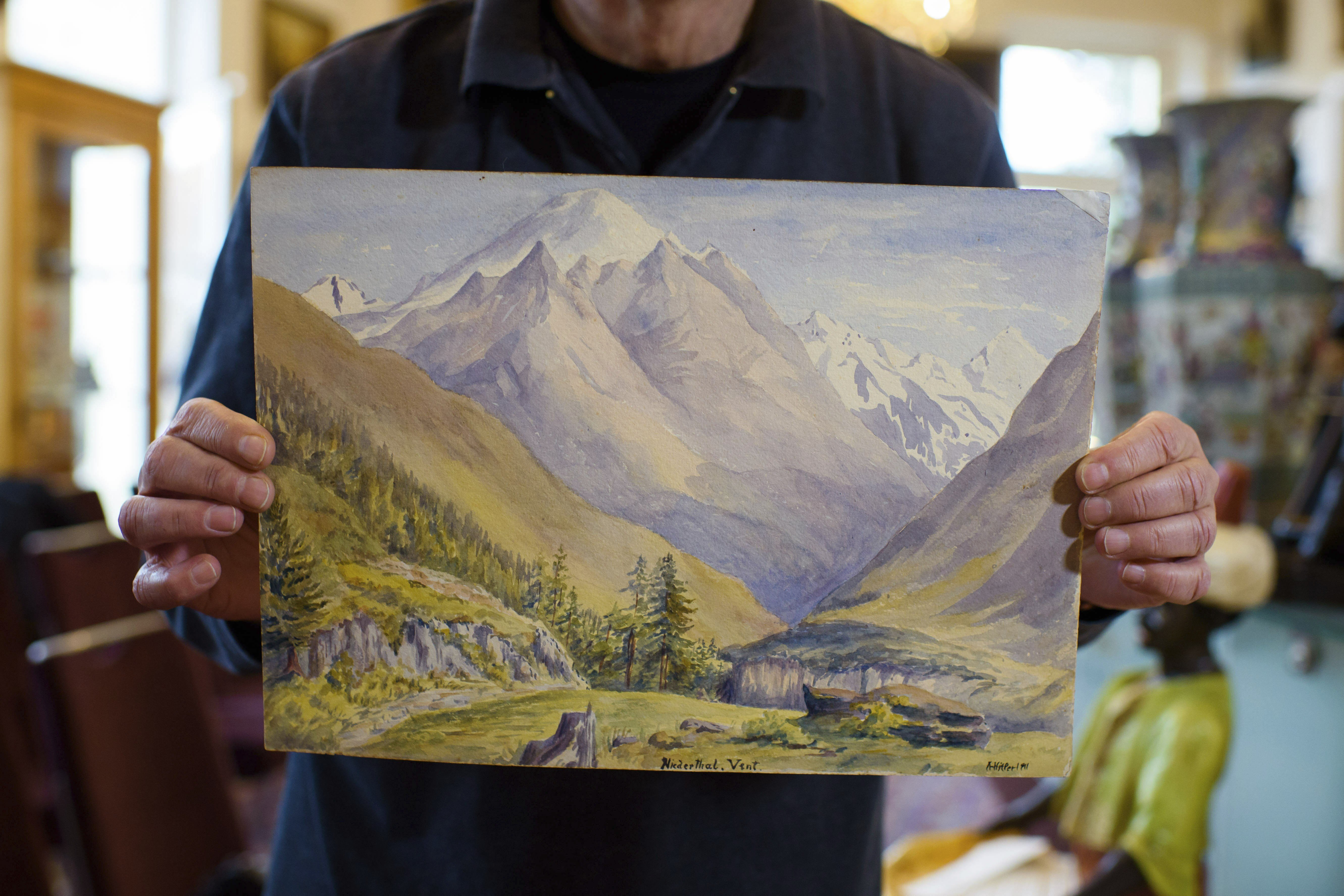In the photograph, a man wearing a dark blue collared shirt is holding up a painting that obscures his face; only his upper body and hands are visible. The painting, gripped on either side by the man's hands, depicts a serene nature scene. In the foreground, green-covered hills and pine trees frame a V-shaped valley, while further back, majestic rocky mountains rise, leading to towering, snow-capped peaks under a sky with a few clouds. The bottom of the painting includes an inscription that reads "hinder that, comma, vent," alongside an undecipherable signature. Behind the man, the blurred background reveals a room filled with large ceramic pots, statues, and other art pieces, including a partial view of an African American figure in a green shirt. Light filters in from windows on both the left and right sides, adding a warm glow to the setting.